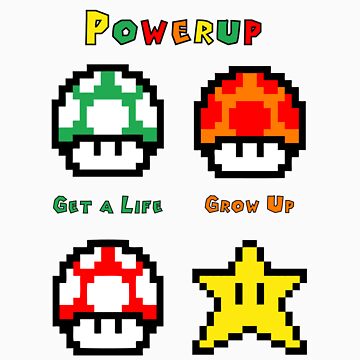The image titled "Power Up" features the text "Power Up" in colorful capital letters, each character in a different color: P in yellow, O in green, W in red, E in orange, R in yellow, U in green, and P in red. Below this vibrant title, two cartoonish Mario game power-ups are depicted side by side. The power-up on the left is a green mushroom with a white pattern on its cap, while the one on the right is an orange mushroom with a red pattern and orange hair. Just below these mushrooms, there is text with contrasting colors: "Get a Life" in green on the left, and "Grow Up" in orange on the right. At the bottom of the image, a red and white mushroom with eyes is placed on the left side, and to its right is a yellow star with two black eyes. The entire composition is presented against a light gray background, with each character and power-up having distinguishable, heavy black outlines.